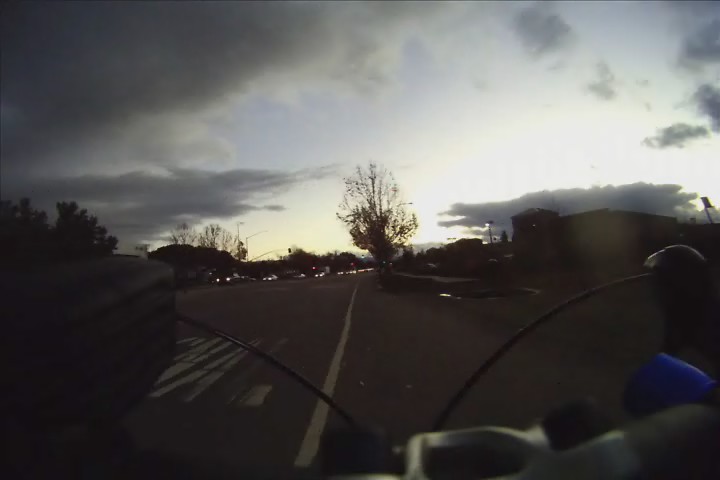In the image, the sky is predominantly filled with a bright white light, yet it is sporadically interrupted by gray clouds situated in the top left and right corners. The horizon is marked by several trees: a prominently dormant tree with bare branches extends its limbs to the left, while further to the left, a leafy tree can be seen. Dominating the foreground is a gray and black ground surface with a distinct white line running through it, along with some visible text. On the left side of the scene, partially obscured but discernible, is an intriguing motorcycle, identifiable through its distinct right side mirror.